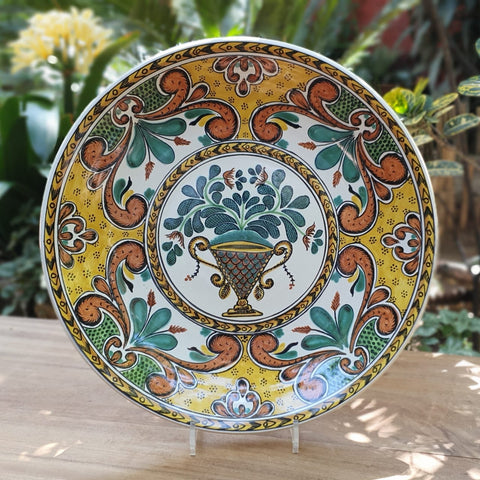This detailed image portrays an ornate china plate positioned upright on a light brown, wooden table, allowing the intricate wood grain to be visible. The picture is taken outdoors, revealing a backdrop of blurred greenery with leaves and a yellow flower in the upper left corner. The plate stands proudly on a holder, ensuring it's displayed vertically. At the heart of the plate, a golden chalice with two curvy handles on each side is prominently featured. This chalice, embellished with red cross-hatching and gray details, has blue-green leaves with red accents emanating outwards. Surrounding this central element is a circular design with gold accents. The outer section of the plate displays repeating patterns of curvy red lines and trefoil-like motifs, each consisting of three green leaves with red stems, emphasizing a sense of growth and nature. The rim of the plate is elegantly trimmed with gold, enhancing its decorative appeal. This fine piece of china, likely meant for display rather than utility, merges detailed botanical depictions with artistic patterns, making it a striking decorative object.